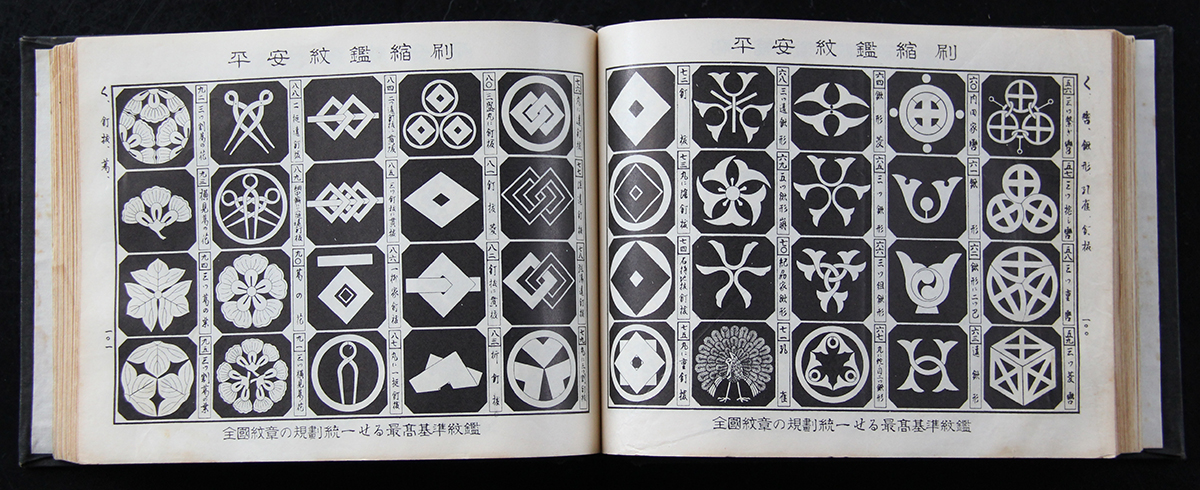The photo captures an open book set against a pitch-black background, with a black cover faintly visible. The book is open to two wide, horizontal pages, each displaying intricate black-and-white geometric designs within a grid of 20 squares, arranged in four rows of five on each page. These designs range from intertwined boxes and upside-down triangles to floral and seashell motifs, all varied and detailed. Above and below the grid on each page, as well as along the sides in vertical lines, are rows of Chinese characters. The pages, appearing to be mid-book, are off-white, suggesting an older or well-used volume dedicated to showcasing these ornate symbols, possibly family crests or emblems.